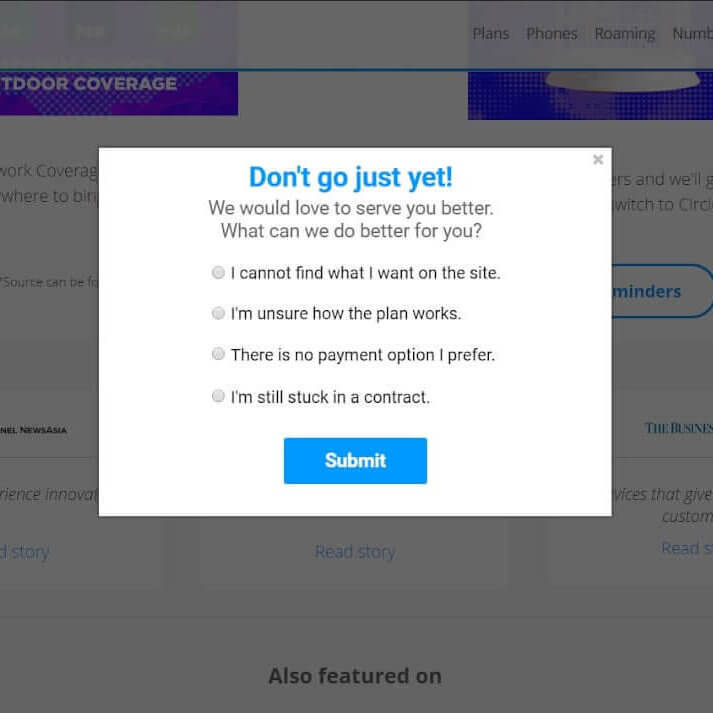The image is a screenshot of a website interface displaying an attempt to cancel a service, likely phone coverage, as suggested by the various labels and options visible. The background features a dark gray color theme with blue and black elements. Readable text on the site includes terms such as "outdoor coverage," "plans," "phones," and "roaming." At the bottom, there are buttons labeled "Also featured on" and "Read Story." 

A significant portion of the image is taken up by a prominent white pop-up box with the headline "Don't go just yet," highlighted in bold blue letters. Below this headline, the pop-up states, "We would love to serve you better. What can we do for you?" This message is followed by four selectable options, each accompanied by a small white button on their left. The options are: "I cannot find what I want on the site," "I'm unsure how the plan works," "There is no payment option I prefer," and "I'm still stuck in a contract." At the bottom of the pop-up, there is a blue rectangular button with the word "Submit" prominently displayed in white letters.